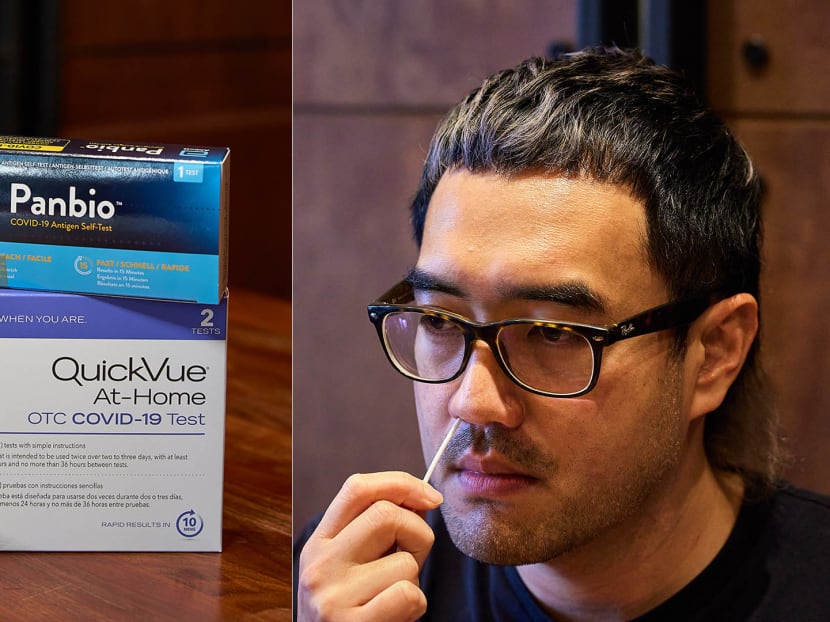This split-screen image consists of two detailed color photographs. On the left, there are two boxes of COVID-19 tests stacked on a wooden table. The top box is labeled "PanBio COVID-19 Antigen Self-Test" and features a dark blue design with a lighter blue stripe at the bottom. Beneath it is a "QuickVue At-Home OTC COVID-19 Test" box, which is medium purple at the top and white on the bottom, with black and purple font detailing that it contains 10 tests and offers rapid results in 10 minutes. The instructions are available in both English and Spanish. 

On the right side of the image is a photorealistic depiction of a young Asian man, likely in his 20s, with short black hair and dark-framed glasses. He is wearing a black t-shirt and has sparse facial hair. The man is performing a self-administered COVID-19 test by inserting a nasal swab into his left nostril with his right hand. He is looking slightly to the left, not directly at the camera.